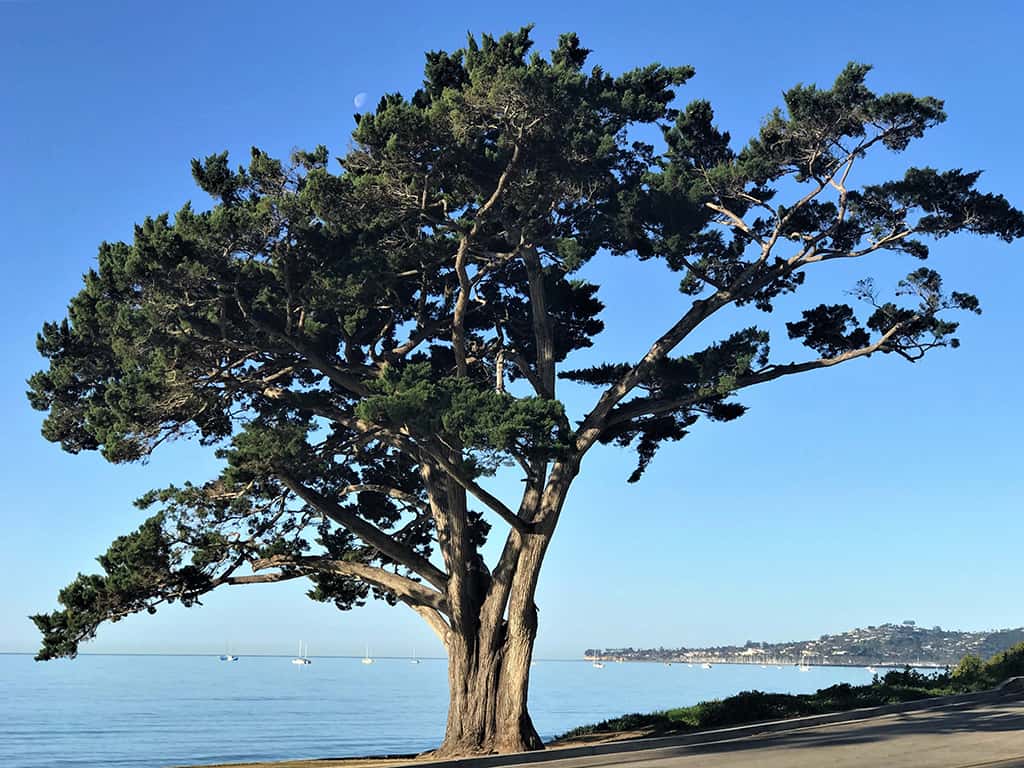This is a brightly lit, natural photograph of a large, ancient cedar or cypress tree with an expansive trunk, approximately three to four feet in diameter. The tree, characterized by its numerous branching limbs, stands prominently near the edge of a large body of water, which might be a lake, ocean, or bay. The clear, cloudless, blue sky serves as a stunning backdrop, with a subtle hint of the moon visible in the daylight. Off in the distance, the serene water is dotted with small sailboats, while to the right, a strip of land extends outward, featuring houses and other buildings. The foreground shows a glimpse of pavement, possibly a parking lot, indicating the proximity to a road. Surrounding the tree, the landscape is lush with green grass and possibly some strawberry plants, contributing to the peaceful coastal vibe, reminiscent of the West Coast, perhaps California.